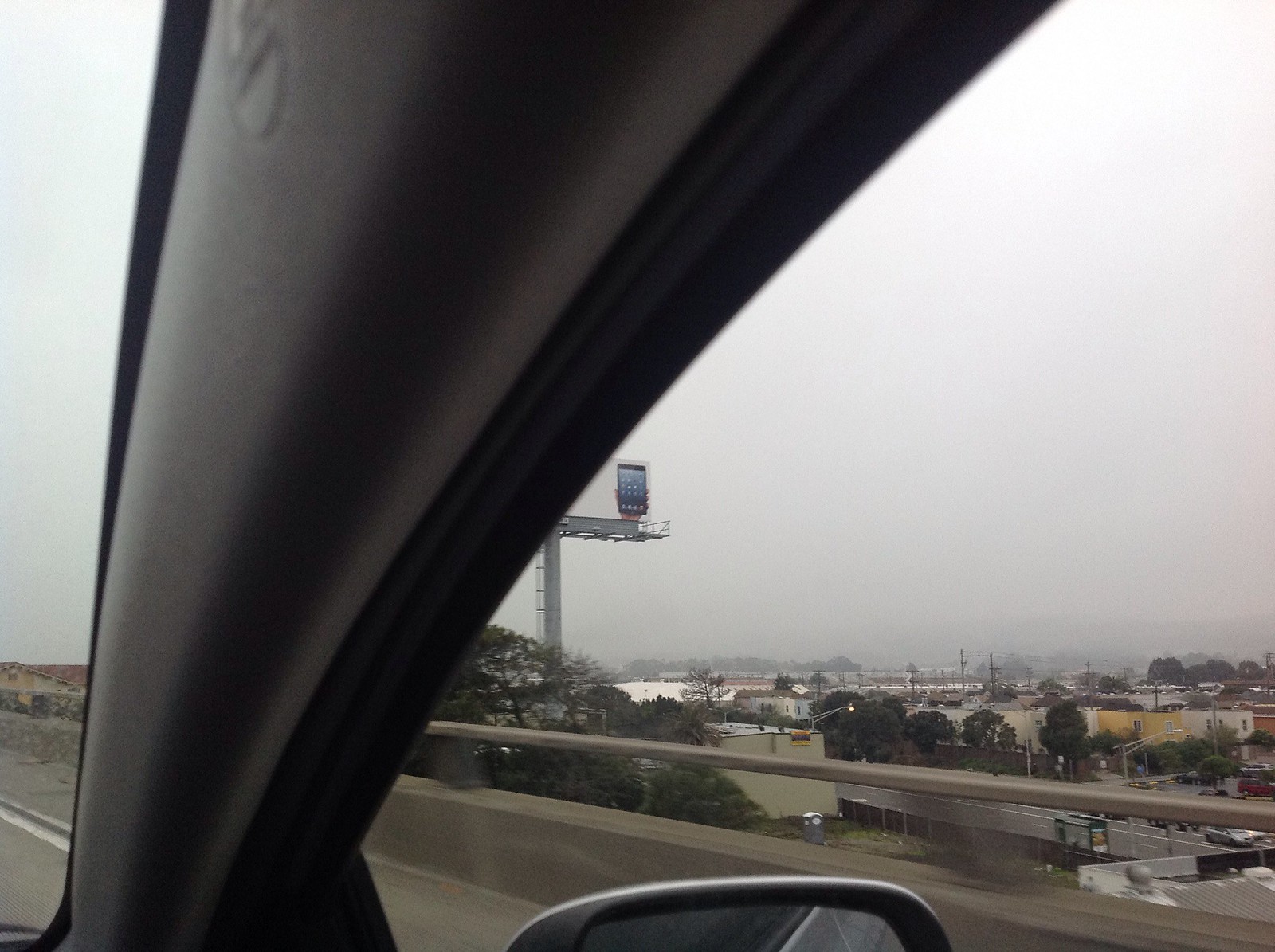This color photograph, captured from the passenger side of a car, appears to have been taken by someone slightly leaning out the window. In the bottom part of the image, the top edge of the car's side mirror is visible. Toward the top left corner, part of the car's interior panel between the dashboard and the window is also seen. This perspective provides a view of the right side of the road, indicating the car is probably crossing a bridge or an overpass. The scene features a concrete wall with a railing, and beyond it, an expansive view of a town or part of a larger city unfolds. The landscape is dominated by numerous trees and residential houses, creating a peaceful, suburban ambiance. The sky overhead is overcast, casting a gray hue over the scene.